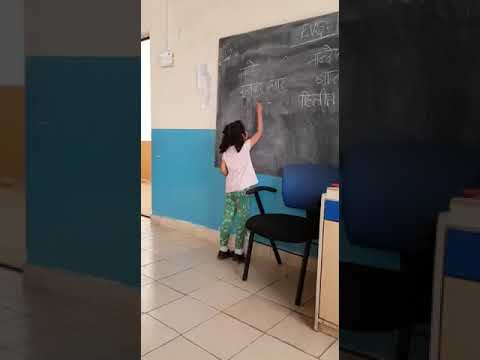The image is a photograph capturing a moment inside a classroom, focusing on a young girl, approximately six to nine years old, standing at the front and writing on a well-worn chalkboard. The chalkboard is heavily marked with white chalk dust and smudges, making its surface appear more gray than black. The writing on the board includes what seems to be an Asian script, although the details aren't distinctly clear. 

The girl, with dark brown hair, is seen from the back. She is dressed in a white short-sleeved blouse, green floral-patterned pants, and black Mary Jane shoes. A blue and black chair and a small cabinet stand beside her. The chalkboard is mounted on a wall that has a blue stripe and beige areas, complemented by white tiled flooring. The scene around her hints at an Indian classroom setting due to the script on the board.

The photograph itself is formatted like a cell phone snapshot. The image is artistically bordered on the left and right by zoomed-in and darker sections of the primary scene, creating a backdrop effect. The left side features an enlarged and faded close-up of the girl, while the right side shows a similar close-up of the cabinet.